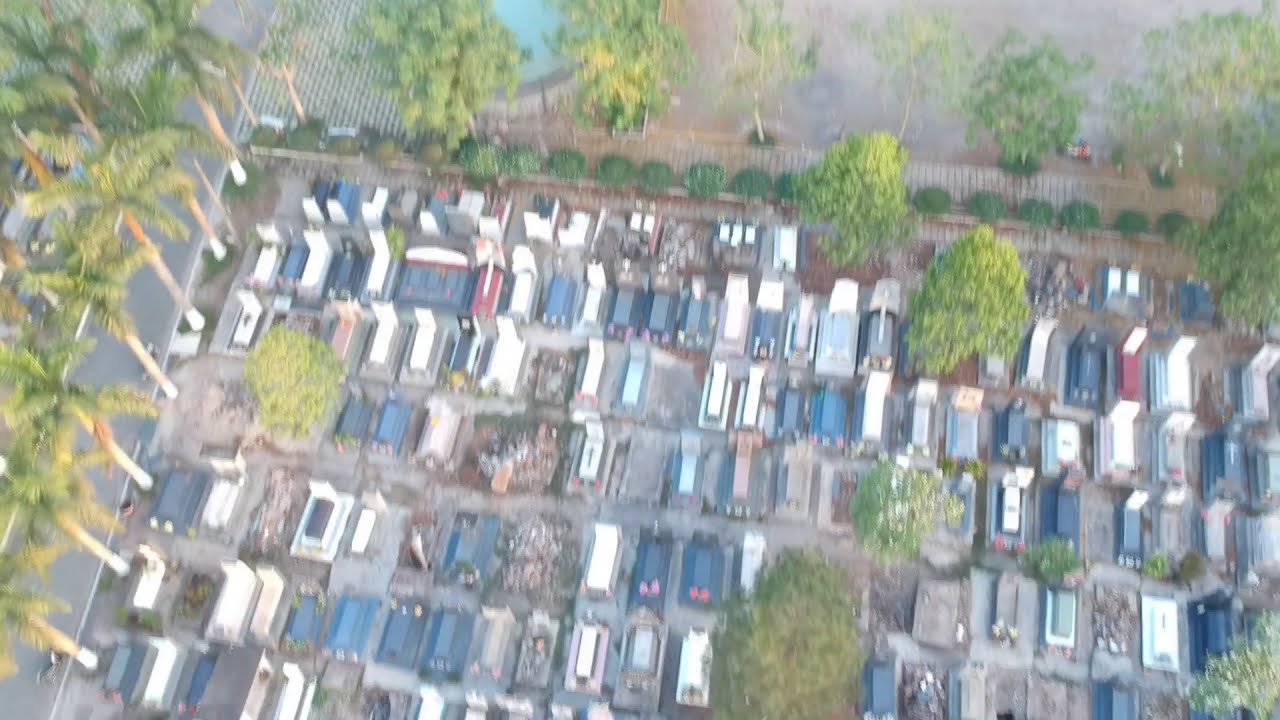This image presents an aerial view of a densely packed housing or trailer park, characterized by rows of small trailer-sized homes. The scene appears to be captured outdoors in broad daylight, showcasing various natural colors such as green from tropical trees and bushes, brown from the dirt ground, and vibrant hues like blue, red, and maroon from the homes. Tropical trees line the edges of the property, enhancing the sense of an organized yet cluttered community. The homes and graves are not centrally aligned but spread unevenly across the frame, with no readable text or numbers present. In addition to the homes, walk paths weave through the area, adding to the structured layout. Despite the blur and distortion in some parts of the image, the depiction is clear enough to suggest a lively, well-lit environment.